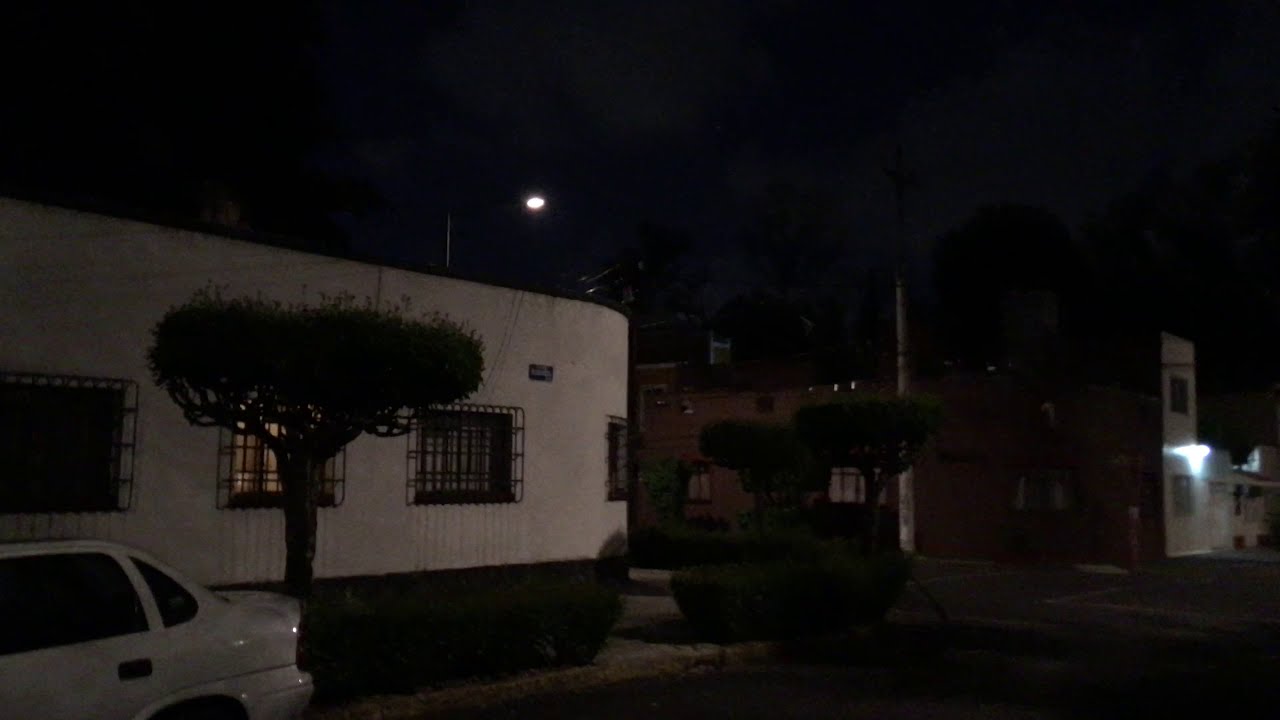The image captures a nighttime street scene characterized by a serene, dimly lit atmosphere. Central to the composition is a single-story white building with three fully visible square windows and a partially visible fourth one, each safeguarded by black bars. In front of this building stands a small tree with a flat, pan-like canopy and nearby, a white coupe with dark-tinted windows, oriented leftward. Positioned on the left side of the scene, this part of the image highlights the intersection of a black asphalt street. 

In the background to the right of this building, stands a taller complex - a light brown two-story building, adjoined by a similar height white building. A streetlight glows softly behind the primary white building, subtly illuminating the scene. Clouds faintly drift across the dark sky, adding texture to the overhead nocturnal expanse. Additional light poles and another light fixture above the entrance of the right-hand white building dot the vicinity, although some remain unlit, contributing to the tranquil darkness that permeates the image.